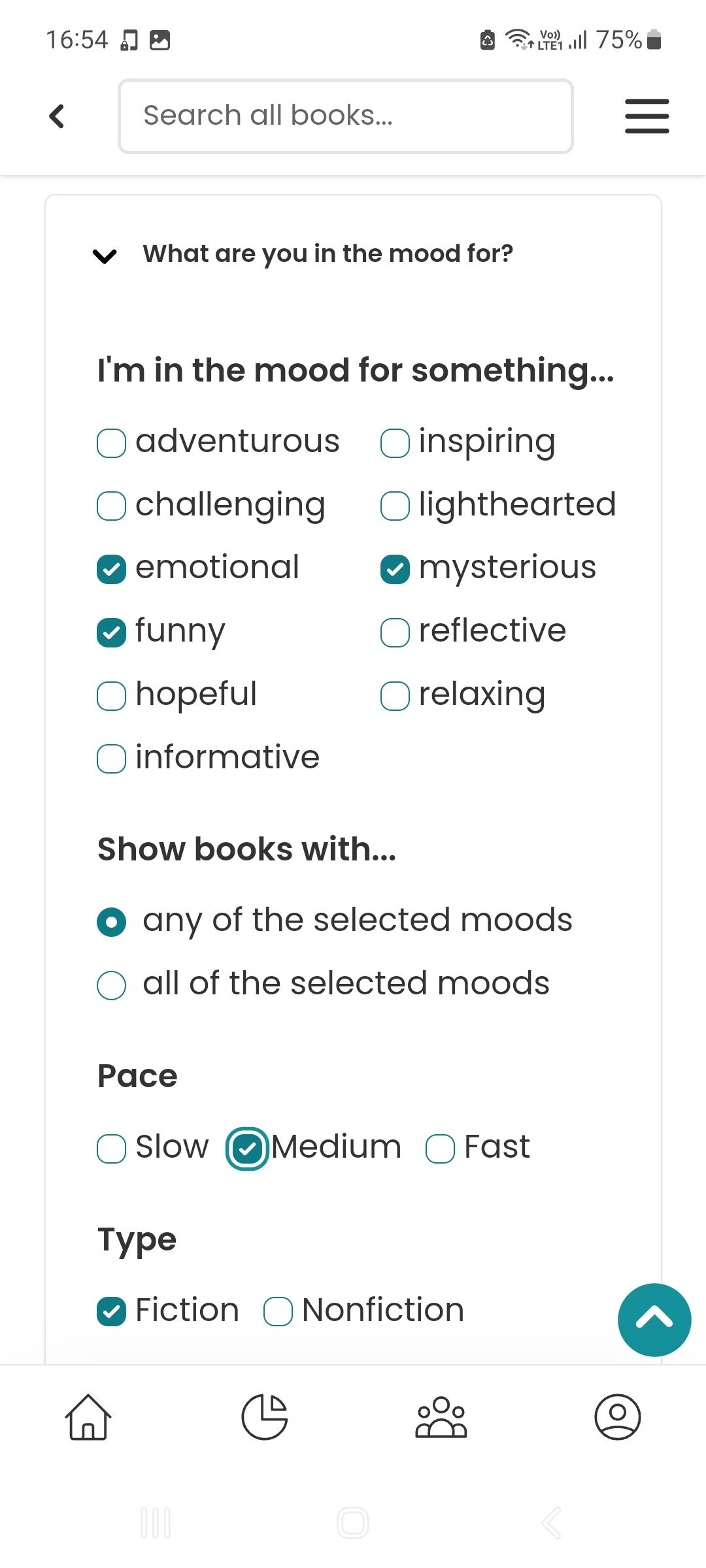The screenshot depicts a mobile phone interface with a white background at the top left corner indicating the time as 16:54. There are two small, unidentified icons next to the time. In the upper right corner, the battery is at 75%, and both Wi-Fi and mobile data are fully connected.

Just below, there's a search bar, represented as a white rectangle with the placeholder text "Search all books..." in gray font. To its left is a left-pointing arrow, and to the right are three horizontal lines, likely a menu icon.

Directly underneath, a larger vertical rectangle displays a drop-down menu titled "What are you in the mood for?" In black font below, it prompts, "I'm in the mood for something..." followed by a list of mood options: Adventurous, Inspiring, Challenging, Light-hearted, Emotional, Mysterious, Funny, Reflective, Hopeful, Relaxing, Informative. The user has selected "Emotional," "Mysterious," and "Funny."

Further down, there is an option to "Show books with..." providing two choices: "Any of the selected moods" (which is selected) and "All of the selected moods" (not selected).

The next section is "Pace," offering "Slow," "Medium," and "Fast" options, with "Medium" selected.

Finally, the "Type" section provides "Fiction" and "Nonfiction" options, of which "Fiction" is selected.